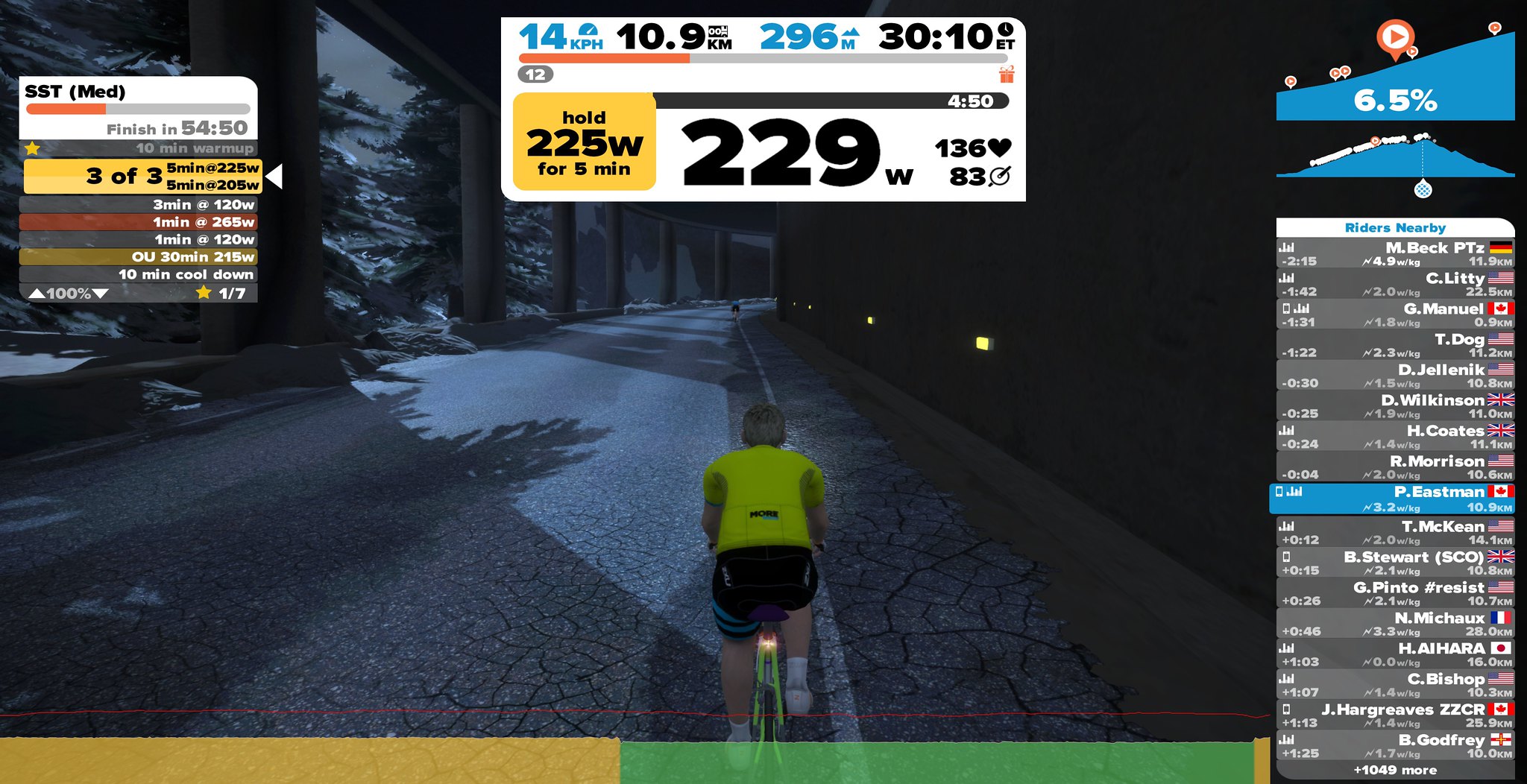The full-color, computer-generated image depicts a nighttime scene in a bicycle simulator showing a biker in third-person view riding on a cobblestone street under an overpass. The biker, who is white, is wearing a yellow jersey, black shorts with blue stripes on the left leg, and white shoes with white socks. To the right of the biker is a concrete wall with yellow lights, and to the left are pillars and trees. In the foreground, a large white box displays various fitness statistics including distance (10.9 kilometers), elevation (296 meters), time (30 minutes 10 seconds), speed (14 kph), heart rate (136 bpm), and power output (229 watts, needing to hold 225 watts for five minutes). Additional boxes to the left and right provide further fitness information and leaderboards, comparing the biker's performance to others from different countries. The upper right corner of the display indicates a 6.5 percent incline on this section of the road.